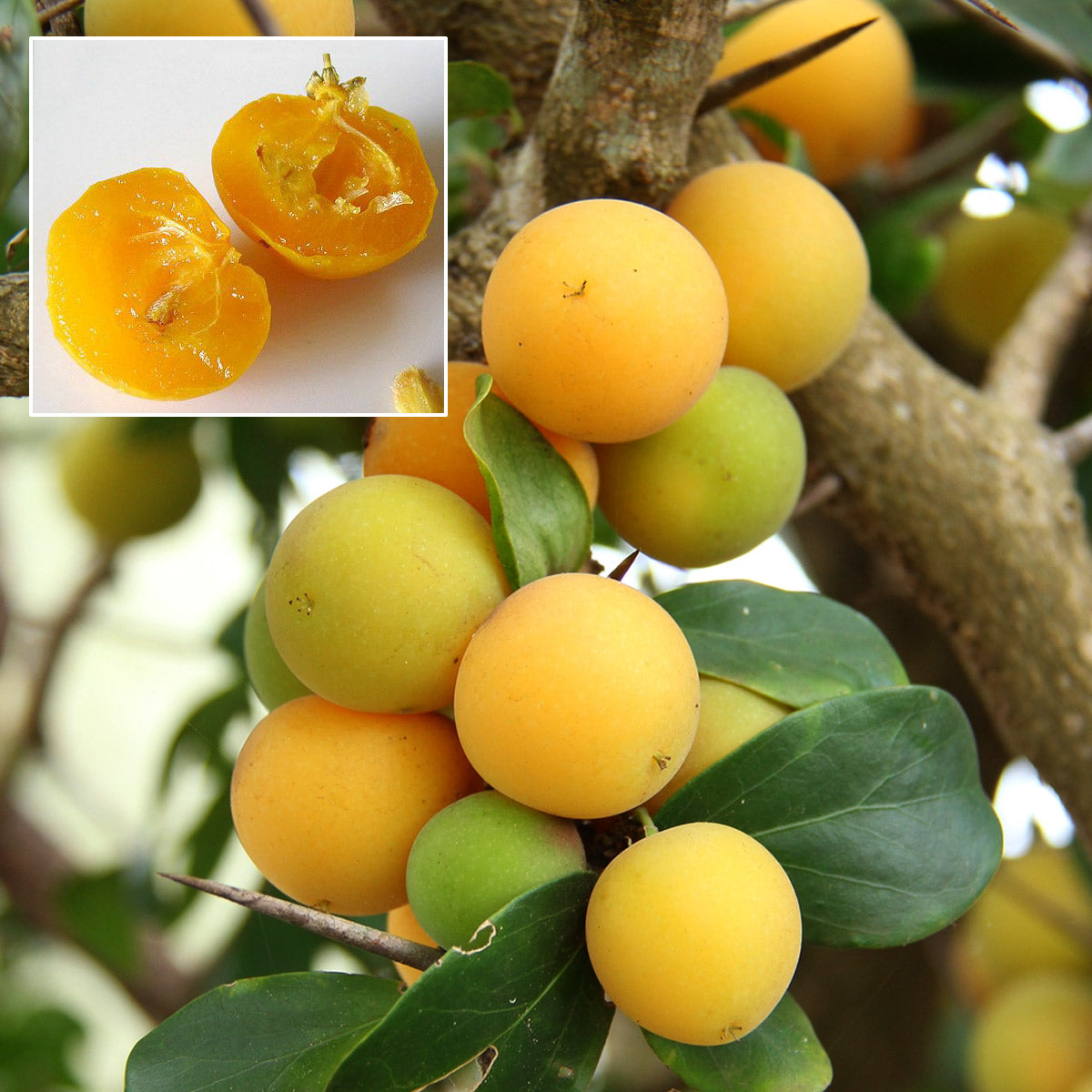The photograph captures a tree laden with an abundance of small, spherical fruits that are transitioning from green to a vibrant orange hue, suggesting degrees of ripeness. Clustered in the center, these fruits exhibit a smooth surface and are set against a backdrop of lush, dark green, waxy leaves. The tree's thick, brown trunk is visible on the right side, extending upwards and adding structure to the composition. To the left, the background appears blurred, with a white, somewhat indistinct sky providing contrast. Adding a specific detail to the scene, an inset square in the upper left corner showcases one of the fruits cut open, revealing its light orange, fleshy interior with a central seed. This detailed portrayal indicates that the fruit is likely a tangerine, despite some ambiguity in identification. The accompanying cut-open view reinforces this speculation, illustrating the appealing, juicy quality of the fruit.